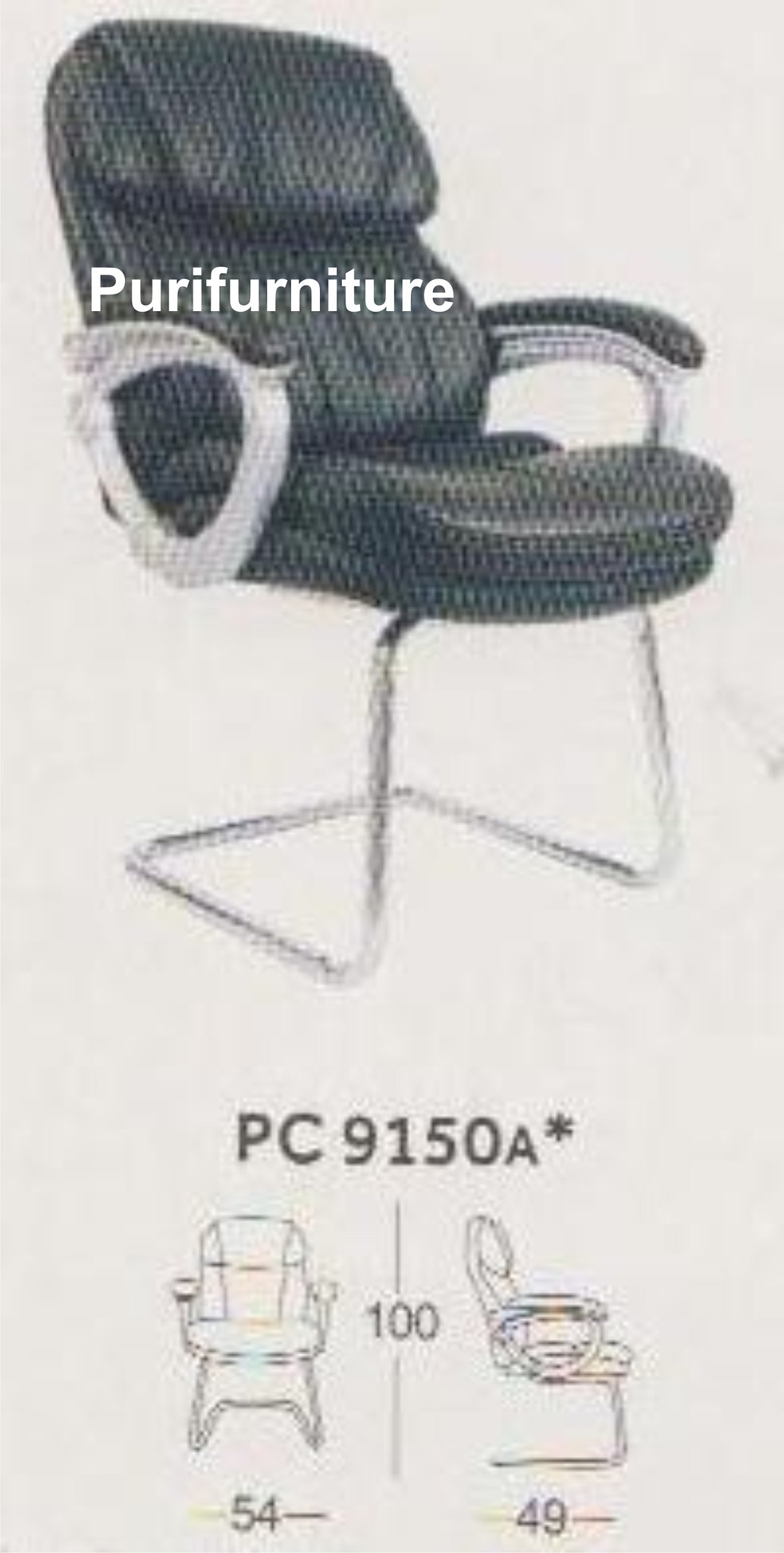This is an image of a sleek, modern desk chair set against a light gray, off-white background. The chair, prominently positioned at the top of the image, features black leather cushions both on the seat and the tops of the armrests, which are supported by gray plastic. Its base consists of unique metal legs that extend downward and then bend outward into a distinctive square pattern, providing support only at the front. Overlaid on this low-resolution image is high-resolution white text that reads "Pura Furniture," emphasized by the stylized spelling "P-U-R-I" in front of "Furniture." Below the chair, in black text, is the model identifier "PC9150A" followed by a small asterisk.

The bottom section of the image contains a sketch-style diagram of the chair, depicting both a front view and a side view, separated by a central vertical line interrupted by the number "100." The front view, positioned on the left, includes a horizontal line marked by the number "54," likely indicating height. The side view on the right features a horizontal line marked "49," probably denoting width. This detailed layout, combined with the precise measurements, suggests the image serves as an advertisement or specification sheet for the chair.